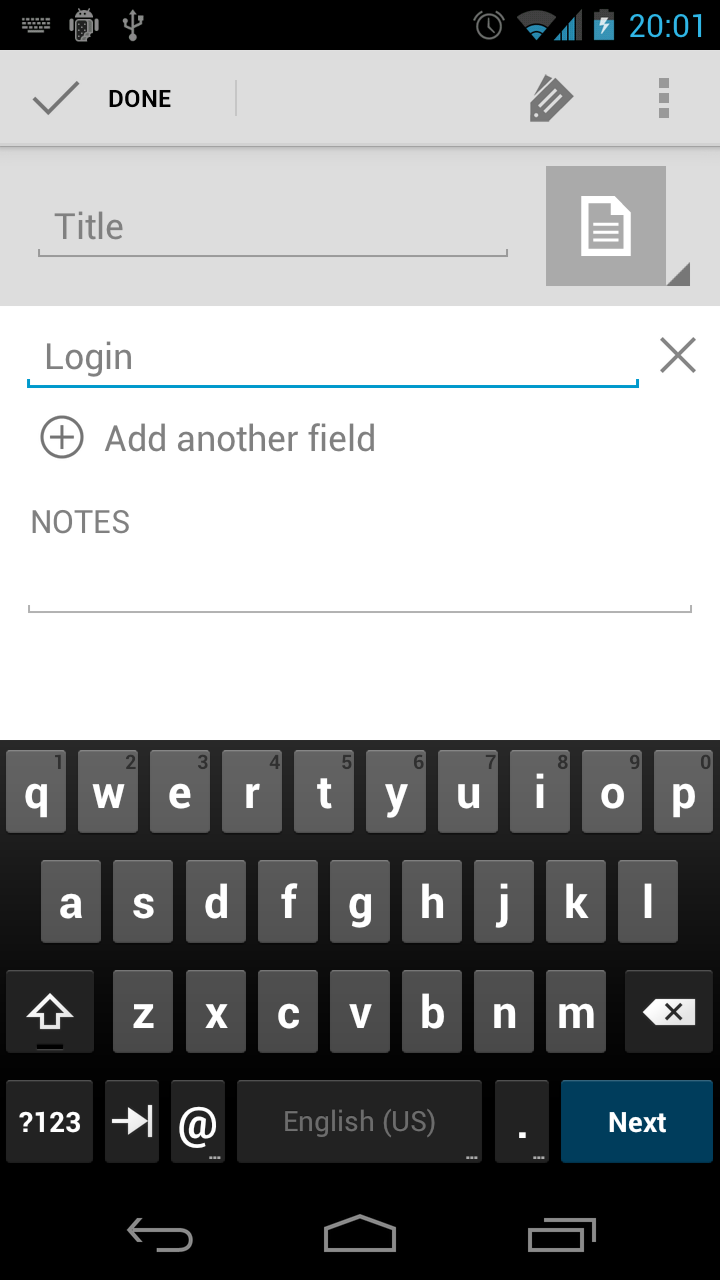The image captures the front interface of a cell phone screen. At the top of the screen is a long, skinny black rectangle displaying several icons, including battery life indicators. Within this area, the time is shown as "20:01" in teal. Below this, there's a section with a gray background featuring a checkmark and the word "Done", accompanied by a floppy disk icon indicating a save function.

Moving further down, there's a section to "Log In", displayed in gray text and underlined with a teal line, ending with a gray "X". Beneath this section is a circular button with a plus sign, labeled "Add Another Field". This is followed by a blank notes section with a gray line indicating where text can be entered.

At the bottom of the screen, the device's keypad is visible. The background of the screen is black, while the keys are gray, and the letters on the keys are white. In the lower right-hand corner of the keypad, there's a prominent teal button labeled "Next" in white letters, indicating progression to the next step.